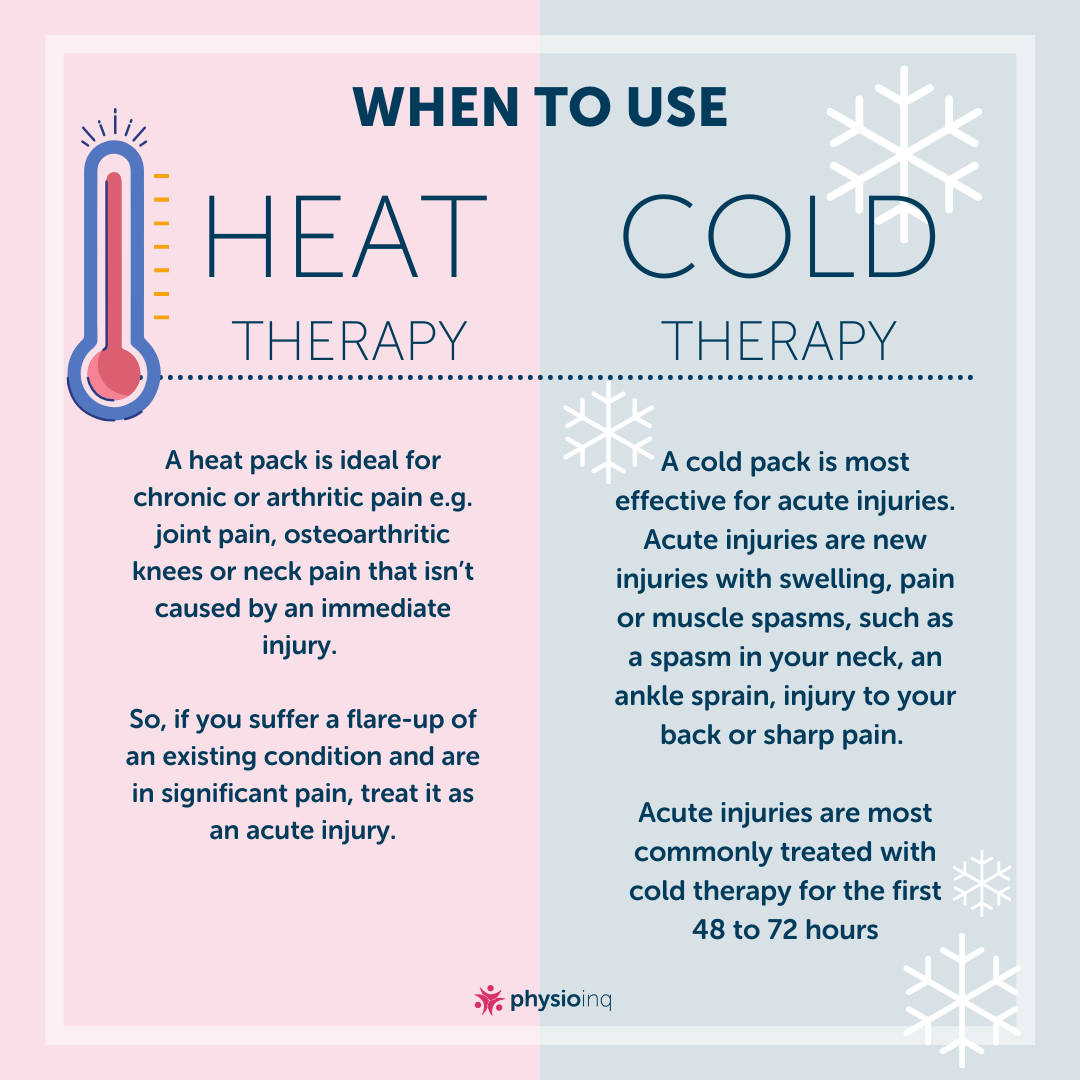This is an instructional leaflet related to physical therapy, produced by Physio INQ. The leaflet provides clear guidance on the appropriate use of heat and cold therapy for pain relief. At the bottom, the leaflet features the Physio INQ logo in navy font alongside a pink icon. The leaflet is visually divided into two sections: one for heat therapy and one for cold therapy.

The heat therapy section, set against a light pink background with navy font, features a red and blue thermometer graphic. At the top, it states "When to Use Heat Therapy". This section explains that a heat pack is ideal for managing chronic or arthritic pain, joint pain, osteoarthritic knees, or neck pain that isn’t caused by an immediate injury. It advises that if you experience a flare-up of an existing condition and significant pain, you should treat it as an acute injury.

The cold therapy section is set against a gray background, also with navy font, and is decorated with white snowflakes. At the top, it says "When to Use Cold Therapy". It explains that a cold pack is most effective for acute injuries, which are new injuries accompanied by swelling, pain, or muscle spasms. Examples include a muscle spasm in the neck, an ankle sprain, a back injury, or sharp pain. The leaflet recommends utilizing cold therapy for the first 48 to 72 hours following an acute injury.